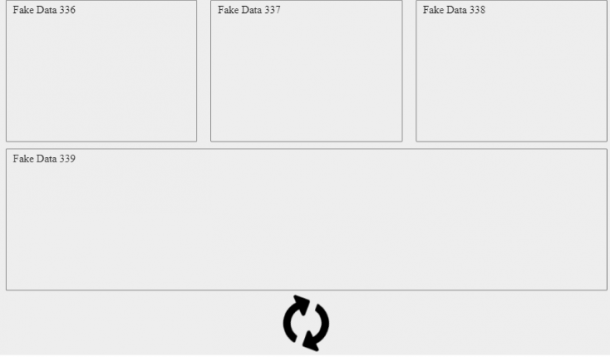The image features a neatly arranged layout with three light gray squares positioned at the top and one elongated light gray rectangle situated beneath them. Each geometric shape bears a label in the top left-hand corner. The labels on the squares from left to right read: "fake data, 336," "fake data, 337," and "fake data, 338." The rectangle below is labeled "fake data, 339." At the very bottom center of the arrangement, there is a refresh icon, depicted by two black arrows forming a circular motion, indicating a reloading action.